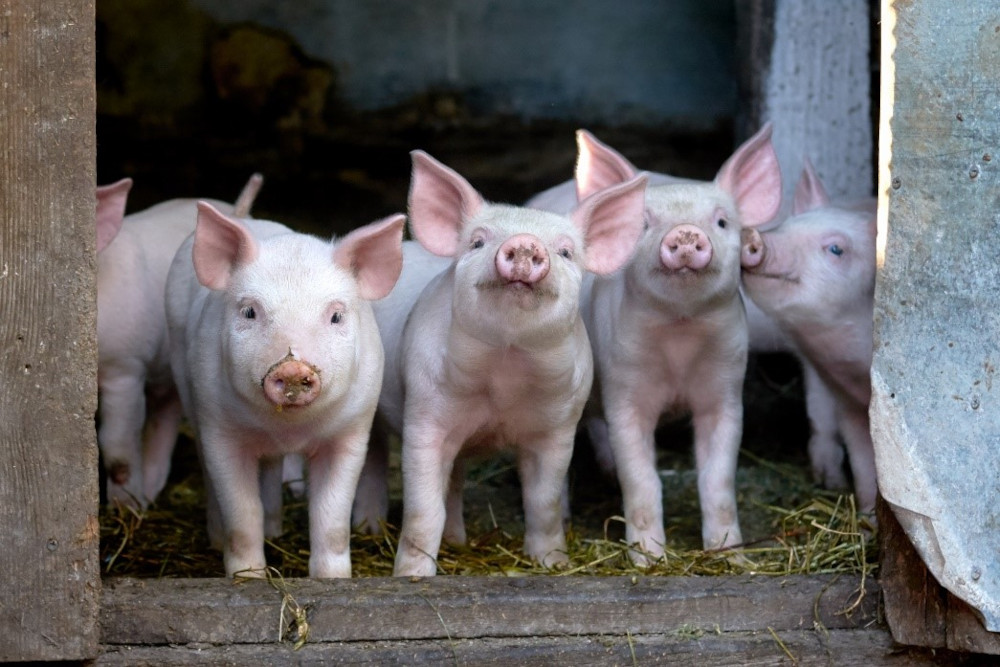In this detailed photograph, we see five young piglets standing close together in the doorway of a wooden shed. Each piglet is characterized by its white body and light pink features, including their ears, snouts, and chests. Their short legs support them as they stand on a floor covered with greenish-yellow straw. The piglets' innocent black eyes, framed by white eyelashes, look curiously at the viewer, with three in the middle making direct eye contact. The piglet on the far right touches its nose to the piglet next to it. The backdrop includes the dim interior of the shed, a doorframe of dark gray and brown wood, and a metal sheet on the right side. The back wall is a mix of dark blue and dark brown, adding context to their rustic environment.